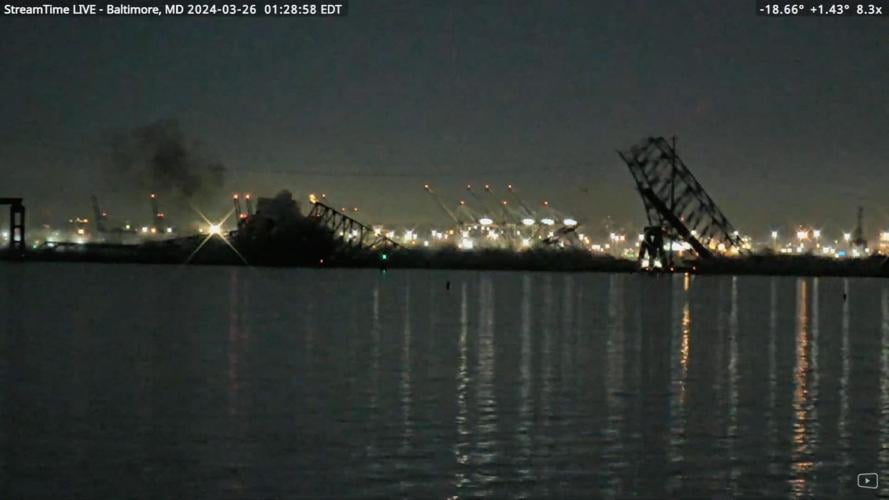This nighttime photograph captures the dramatic collapse of the Baltimore Bridge, taken on March 26, 2024, at 1:28 AM Eastern Time, as indicated by the text at the top that reads "stream time live, Baltimore, Maryland, 03-26-24 01:28:58 EDT." The image appears to be a screenshot from security camera footage positioned across the river, displaying the seaport and shipping area of Baltimore in the distance. The collapsed bridge is shown in two pieces with large sections jutting out of the water and others hanging precariously from support struts. Thick black smoke rises on the left side of the image, adding to the scene's intensity. In the background, numerous lights, perhaps from buildings or ships, illuminate the skyline and reflect off the dark waters in the foreground. Additional onscreen data includes the coordinates (-18.66 degrees, +1.43 degrees), and a zoom level marked as 8.3X, adding to the archival and dramatic nature of the scene.